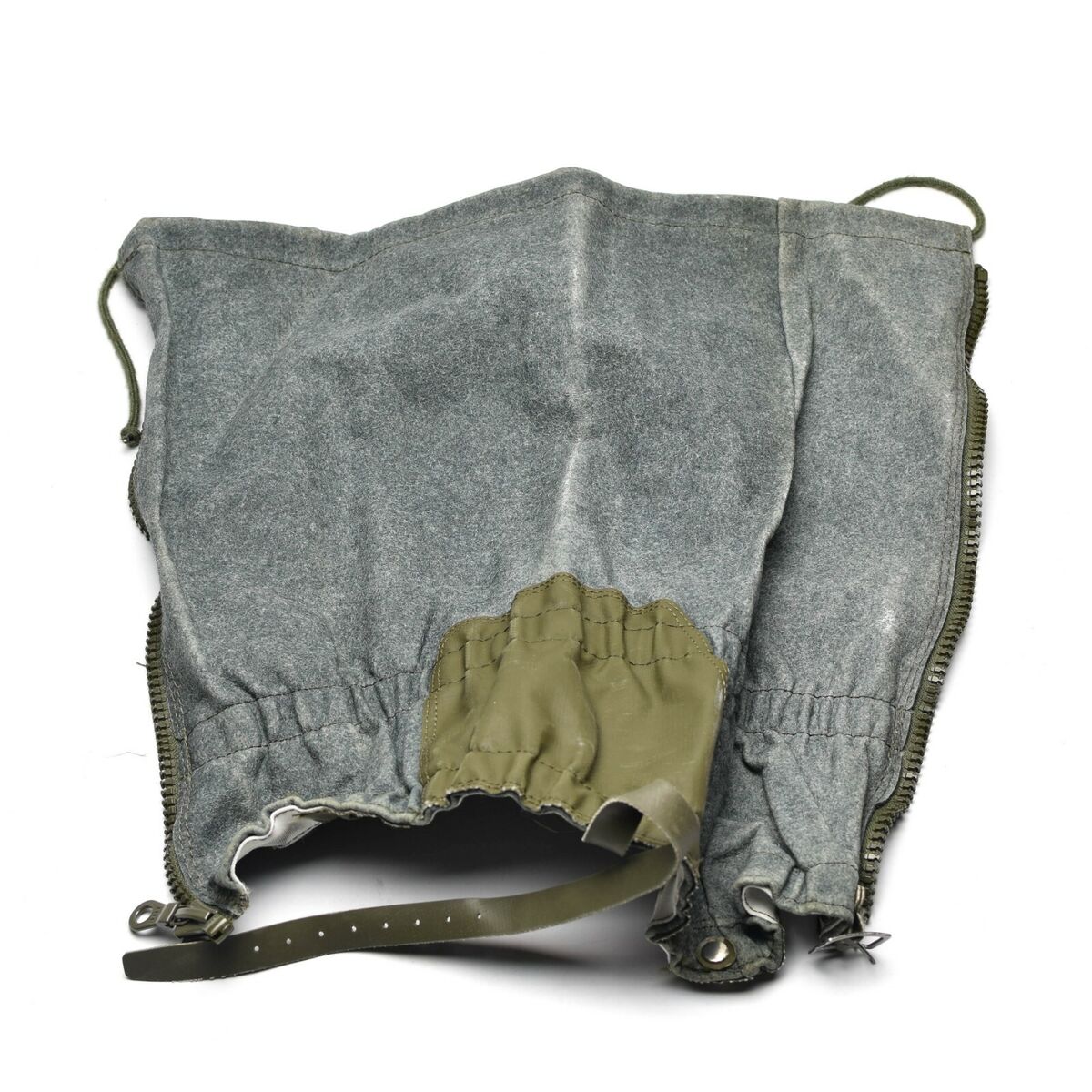The image showcases a grey denim garment set against a white background. The garment appears to be a type of jacket or potentially a sack or small skirt, featuring a distinct jacket-like texture. Notable details include zipper mechanisms on both the left and right sides, which are colored green. The zipper tab is located at the bottom left. The garment also sports a gray elastic band towards the bottom, creating a cinched or pinched effect with parallel stitching. There is a leather strap emerging from the lower part and a noticeable pull string at the top, with strings extending from both the upper left and right sides. Additionally, there’s a brown, almost circular spot toward the waistband, which is situated at the bottom of the image. The garment also includes a belt-like object within the center where the button next to the zipper would typically be. Overall, the piece has outdoor wear characteristics, potentially serving as a multifunctional clothing item.